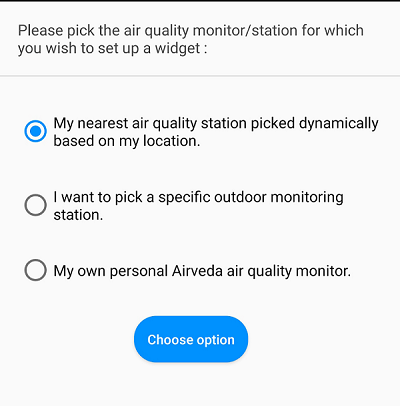A web page for selecting an air quality monitoring station is displayed. The header reads "Please pick the air quality monitor/station for which you wish to set up a widget." Below the header, there are three options for users to choose from. The first option, which has been selected, is labeled "My nearest air quality station picked dynamically based on my location." This selection is indicated by a small blue solid circle within a white circle, enclosed by another blue outlined circle. 

The second option is "I want to pick a specific outdoor monitoring station," while the third option is "My own personal Airveda (A-I-R-V-E-D-A) air quality monitor." Below these choices, there is a blue button labeled "Choose option." The user has opted for the dynamically selected nearest air quality station, but the purpose for this selection is not specified.